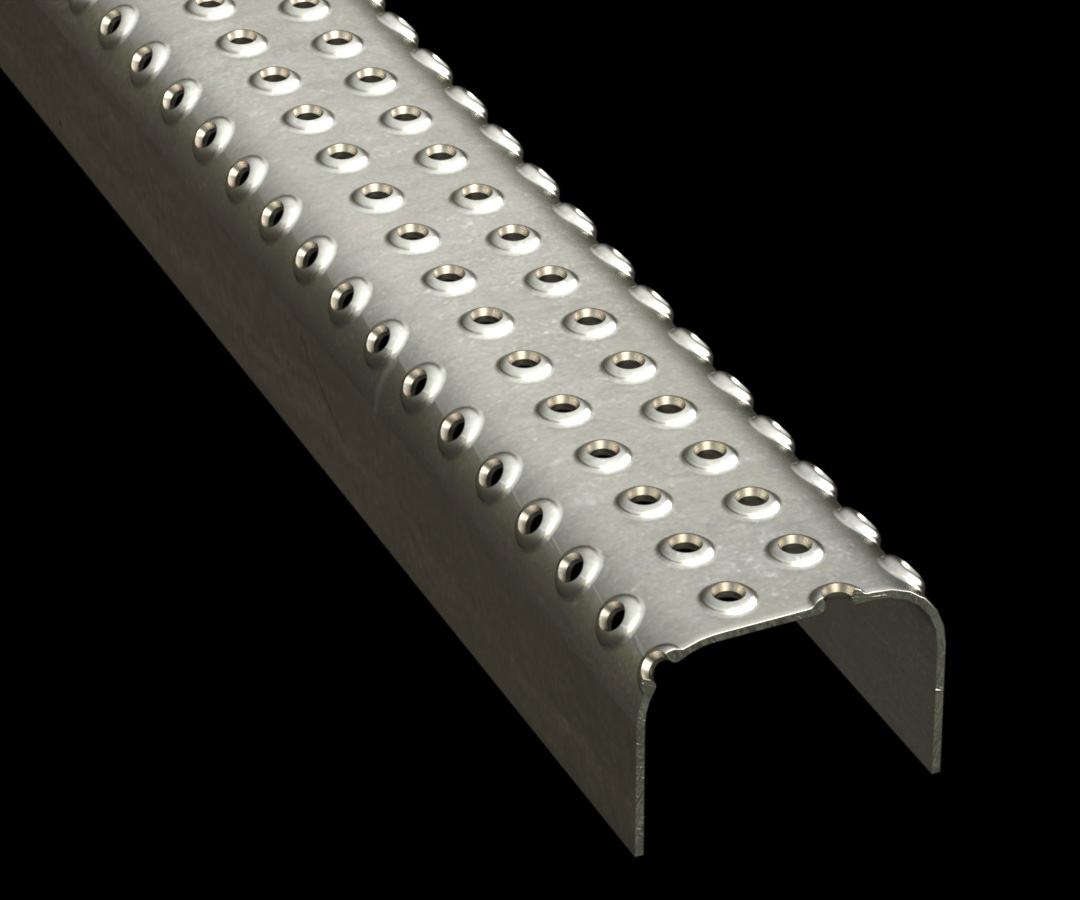This detailed close-up photo showcases a thin, polished silver metal bar, smoothly bent into a shape resembling a lowercase 'n'. The bar is punctured with four orderly rows of small holes, each approximately half an inch apart. The solid, featureless black background emphasizes the bar's sleek, professional presentation, highlighting its reflective quality without creating distracting highlights. The metal component appears to be part of a machine, meticulously captured with professional lighting for a refined, product-like appearance.